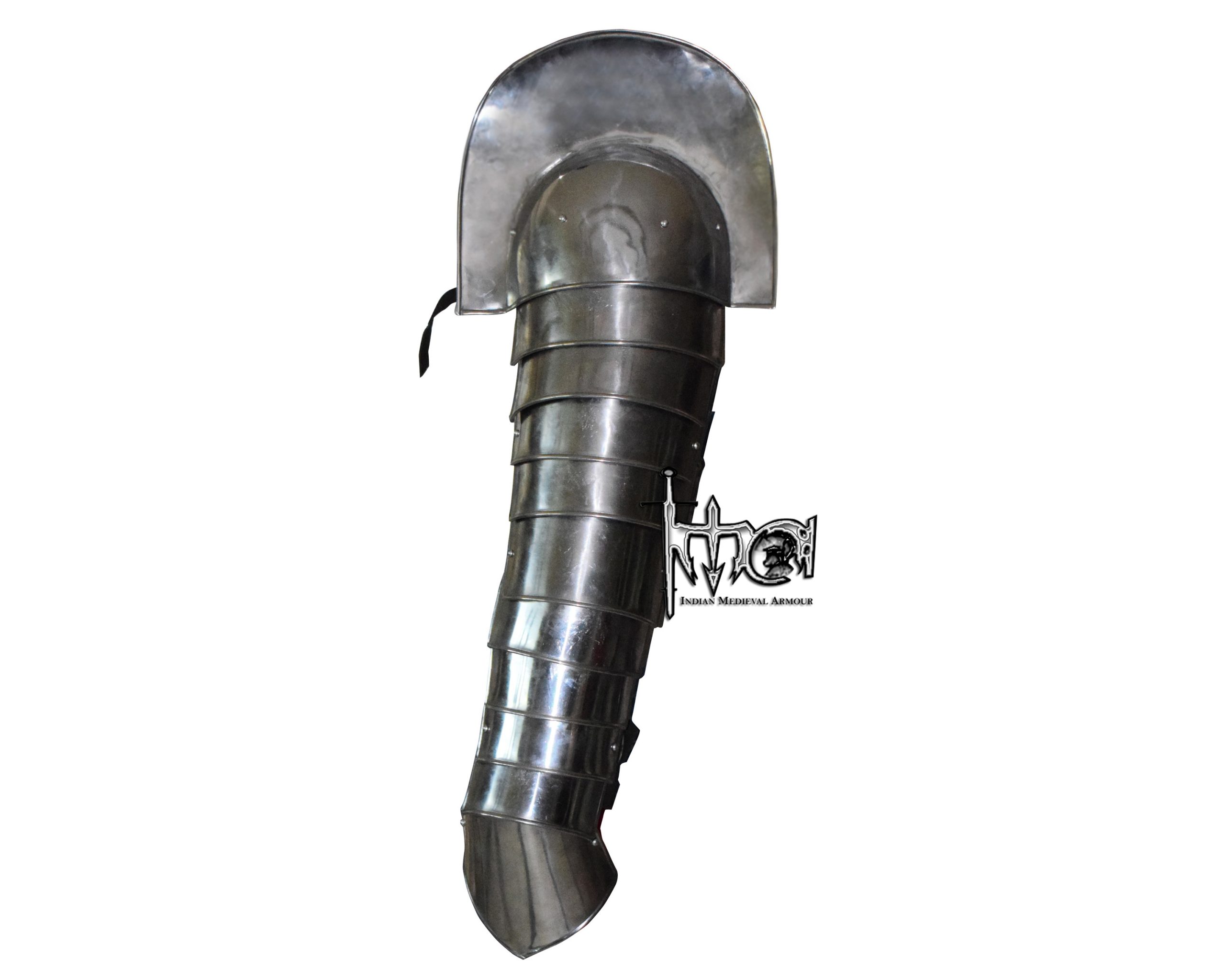The image depicts an item that resembles a piece of medieval armor, specifically designed to protect an arm. The item features a series of layered, shiny gray metal bands that create an appearance similar to an elephant’s trunk or a gas nozzle, extending from what might be a shoulder piece down to the wrist. The metal glistens under the light, highlighting its polished, silver-like surface. In the center of the image, there is a logo that reads "Indian Medieval Armor," which could indicate the item's historical style or brand. The photograph is set against a plain white background, making the details of the metalwork and design stand out clearly.